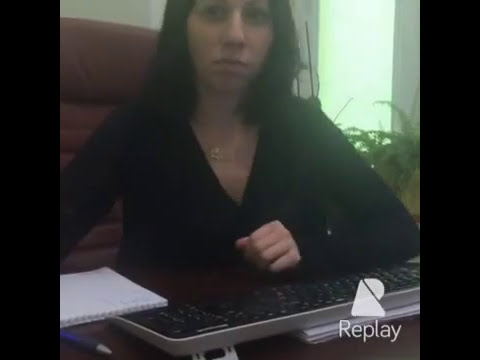In this detailed image, a woman with shoulder-length dark brown hair is seated at a wooden desk with a dark brown finish. She is wearing a bluish-purple long-sleeved V-neck shirt, along with a visible necklace. The woman is centered in the image, sitting in a cushioned light brown chair, and is looking slightly to the side rather than directly at the camera, without a smile. 

On the desk, positioned in front of her, is a keyboard. To her left, there is a blue pen and a notebook, while her left arm and hand are visible resting on the desk. The setting appears to be a home office, as indicated by the indoor environment with daylight streaming through a window on the right side of the image. Near the window, there is a green plant contributing to the warm atmosphere. Also, slightly visible are what seem to be drapes and a wall behind her. The overall color palette includes off-white, brown, black, tan, blue, gray, silver, green, and lime green.

Finally, in the bottom right corner of the image, there is a logo that resembles a filled-in letter "R" with the word "replay" beneath it, indicating perhaps the context or purpose of the image. The photo is taken at a slight angle, helping to capture the various elements in the scene.